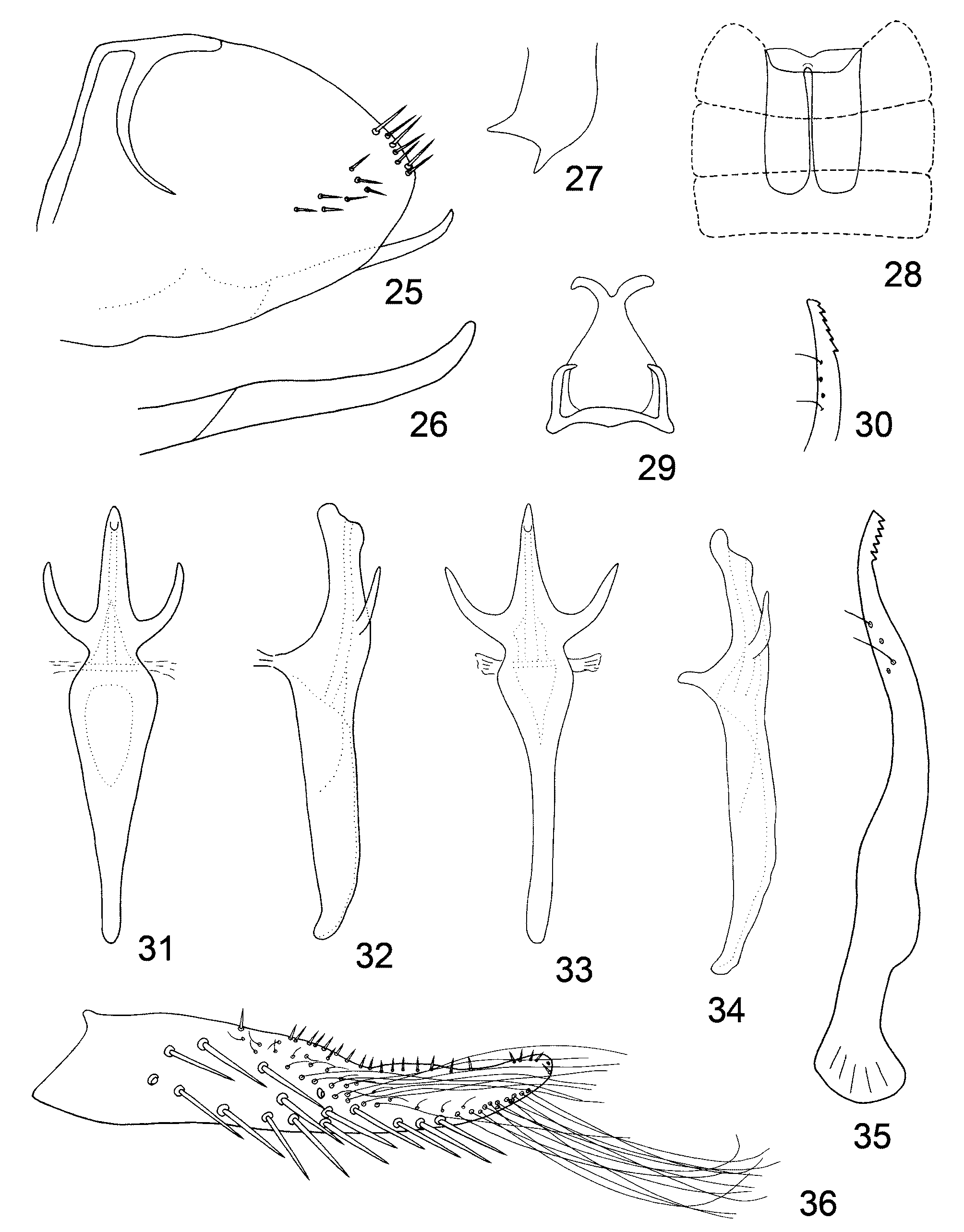The image features a black and white print, potentially drawn by hand, showcasing various labeled shapes and figures which appear to be schematics of animal parts. Starting from the top left, figure number 25 depicts half of a backward "C" adorned with fine hairs, some of which lay flat on its surface. Directly below, figure 26 resembles a slender, elongated "V" tipped to the right. Moving back to the top, figure 27 is a shape tapering down to a point, then extending right before curving back upward.

Figure 28 comprises two adjacent half-capsules, with dotted lines extending from their tops, moving outward and downward, intersecting through the center. Figure 29 resembles the top of a turnip, while figure 30 is an upside-down "V." The sequence continues with figures 31 to 35, each featuring three tine-like protrusions. At the bottom, figure 36 resembles an arm of a starfish, complete with small pointy extensions and wispy, hair-like strands.

Although the exact nature of the creature these parts belong to remains unclear, it is likely microscopic, given the intricate details and labeling from 25 through 36. The artistic execution of these schematics, potentially made with markers or pens, emphasizes the scientific examination of these enigmatic animal components.